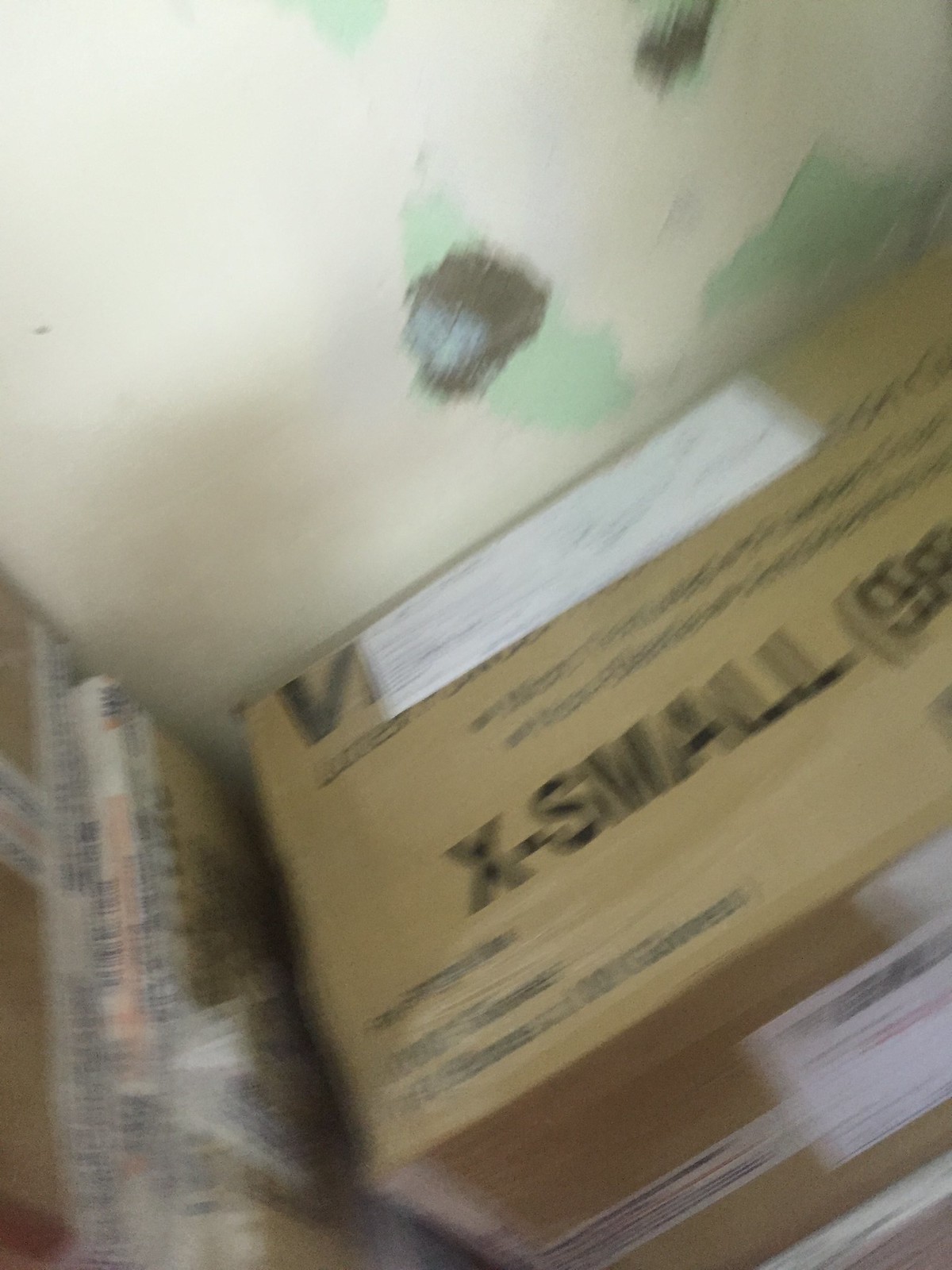This vertical digital photo appears to have been taken accidentally or in a hurried manner, evident from its blurry and angled composition. It shows a collection of tan cardboard boxes on the floor positioned at a 45-degree angle against a wall. The image seems to have been taken from above at an approximately 45-degree downward angle. The wall itself is white but marred by a black smear and patches of green paint. Areas of the wall's previous unsightly brown color are also visible, hinting that this might be a utility or back room with old, chipped paint.

The image's motion blur makes it difficult to discern fine details. One prominent box is partially readable, displaying the text "X-small" in large print, alongside some barely distinguishable numbers and text due to the blurriness. This box also has a white envelope on top and white labels on its side and bottom, with one of the labels featuring a barcode. To the left of this main box, there are additional folded or stacked cardboard boxes, similar in appearance but also out of focus. The overall scene is one of disarray, suggesting a workspace or storage area filled with packaged items awaiting further action.